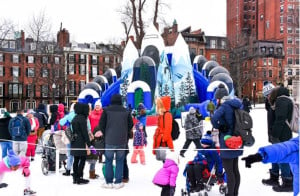The image depicts an outdoor winter scene in a city, possibly New York, Boston, or a city in the UK, featuring a snow-covered ground and large brownstone buildings with a tall building and homes in the background. Central to the photograph is a roped-off, child-like playscape, likely an inflatable castle, adorned with features like fake trees and hoops, and possibly used as a slide attraction. This playscape seems to be drawing significant interest, with numerous adults and children gathered around. The crowd includes kids dressed in strollers with bright winter attire—one in a bright pink coat and white hat, another in a blue hat and jacket—alongside parents and other adults in winter coats. The overall scene suggests a festive atmosphere, possibly around Christmas, though there are no explicit holiday decorations visible.